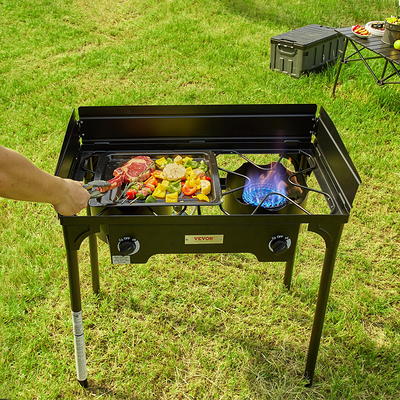The image captures an overhead and slightly downward view of a backyard scene centered around an outdoor black grill. The grill, reminiscent of a gas range with a matte, semi-glossy finish, stands securely on four slender, post-like legs; the front left leg distinguished by white tape wrapped around the bottom. The grill's thin, clover-shaped frame includes a black metal sheet surface on the left side, upon which various fruits, vegetables, and several pieces of beef are being grilled. The right burner, emitting a bluish-purple flame, remains unoccupied. Two control knobs, one for each burner, are visible on the front of the grill, along with a middle tag featuring red text. 

In the top right corner of the image, a small black table with black legs holds a bowl of bright orange and red slices, a white bowl filled with black contents, and a little green pot with yellow plants sprouting from it. To the left of this table sits a thick, black luggage case with green sides. The grill-led food is being attentively turned by a pair of tongs held by an arm extending from the left side of the screen, visible from the elbow down.

The entire setup rests atop lush green grass, interspersed with patches of dried, brownish-tan areas, amplifying the backyard setting's vitality.